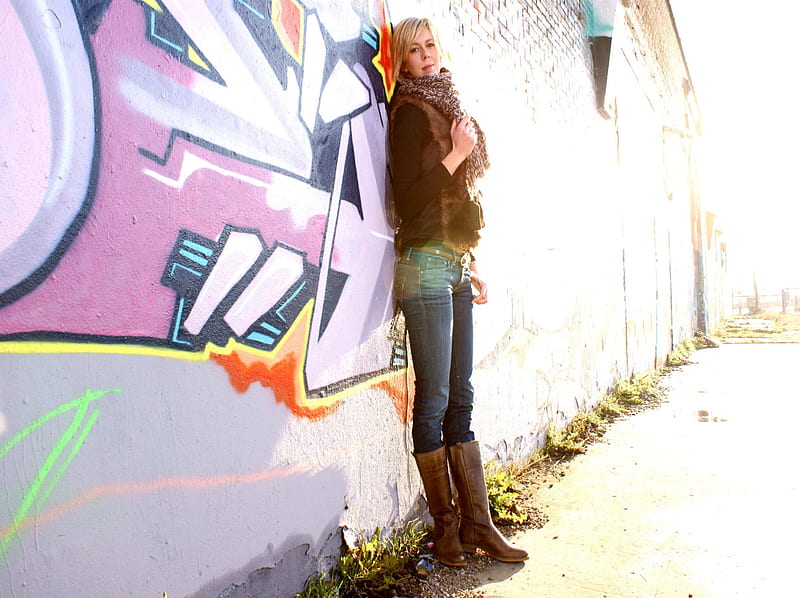This photograph captures a younger Caucasian woman standing against a brick wall adorned with vibrant graffiti in shades of purple, orange, green, and black. The wall appears poorly maintained and fades to white under the intense sunlight illuminating the right side of the image. The woman, who has dark brown hair with blonde highlights, is looking directly at the camera over her right shoulder with a smile. She is dressed in a long-sleeved brown shirt layered with a fuzzy, fur vest, blue jeans, and brown leather boots. She also sports a cheetah-like bandana around her neck. The high contrast of the image emphasizes her figure against the urban backdrop of the alleyway.